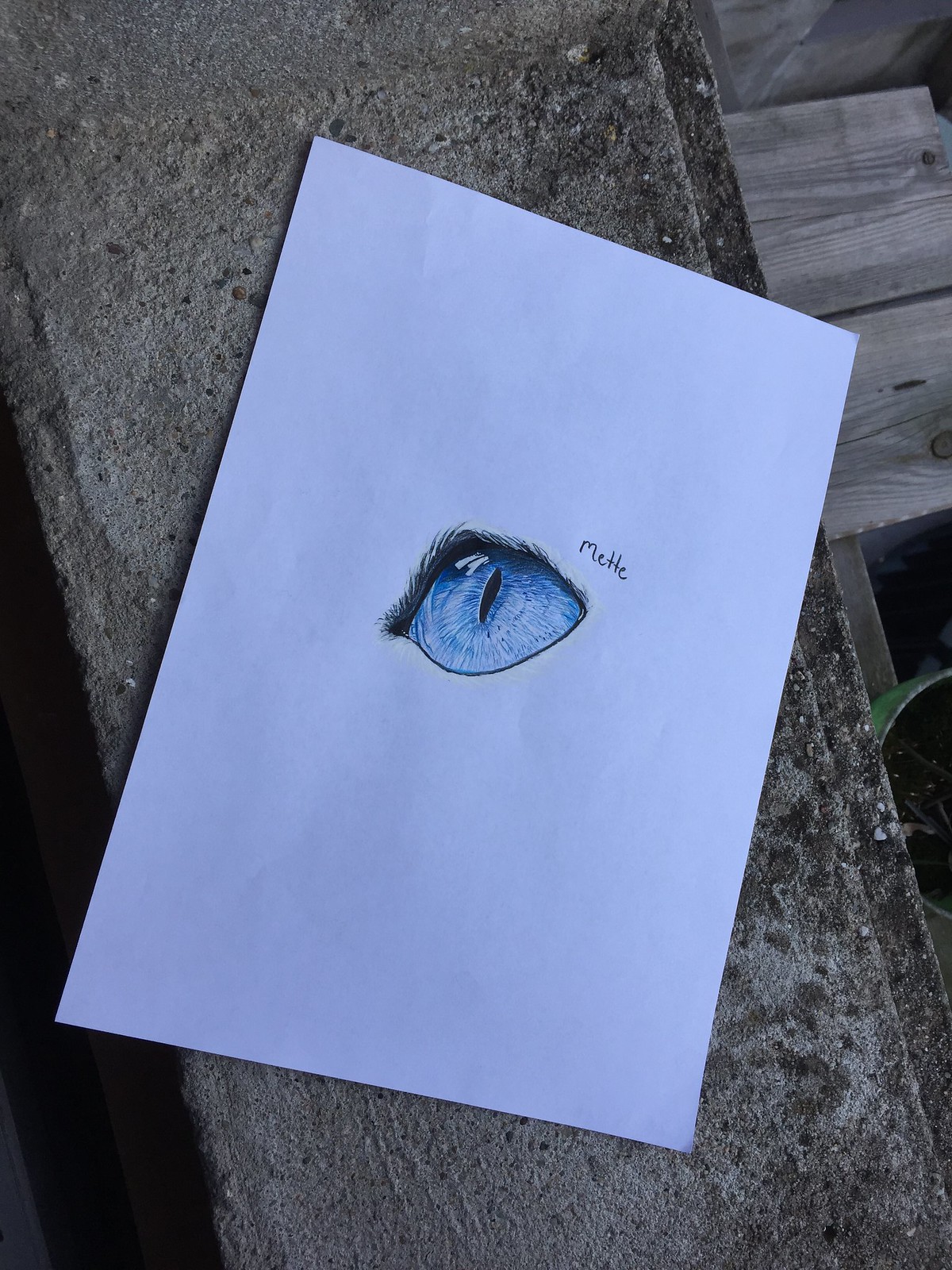The image depicts a detailed, angled view of a white piece of paper resting on a gray concrete barrier. The paper is slightly oriented to the right and features a striking, realistic sketch of a blue almond-shaped eye, centered on the page with its pointed tip facing right. This eye, possibly belonging to an animal, has a distinctive black vertical slit for a pupil and fine, closely-set eyelashes. Above the eye, the name "Medi" is inscribed in pencil. The concrete slab appears to be part of a barrier or walkway, and in the background, there are slats of bleached wood, possibly from wooden steps, visible in the top left corner. The eye is encapsulated by subtle details, such as white bands suggesting highlights and a hint of black fur along the top edge, enhancing its lifelike appearance.